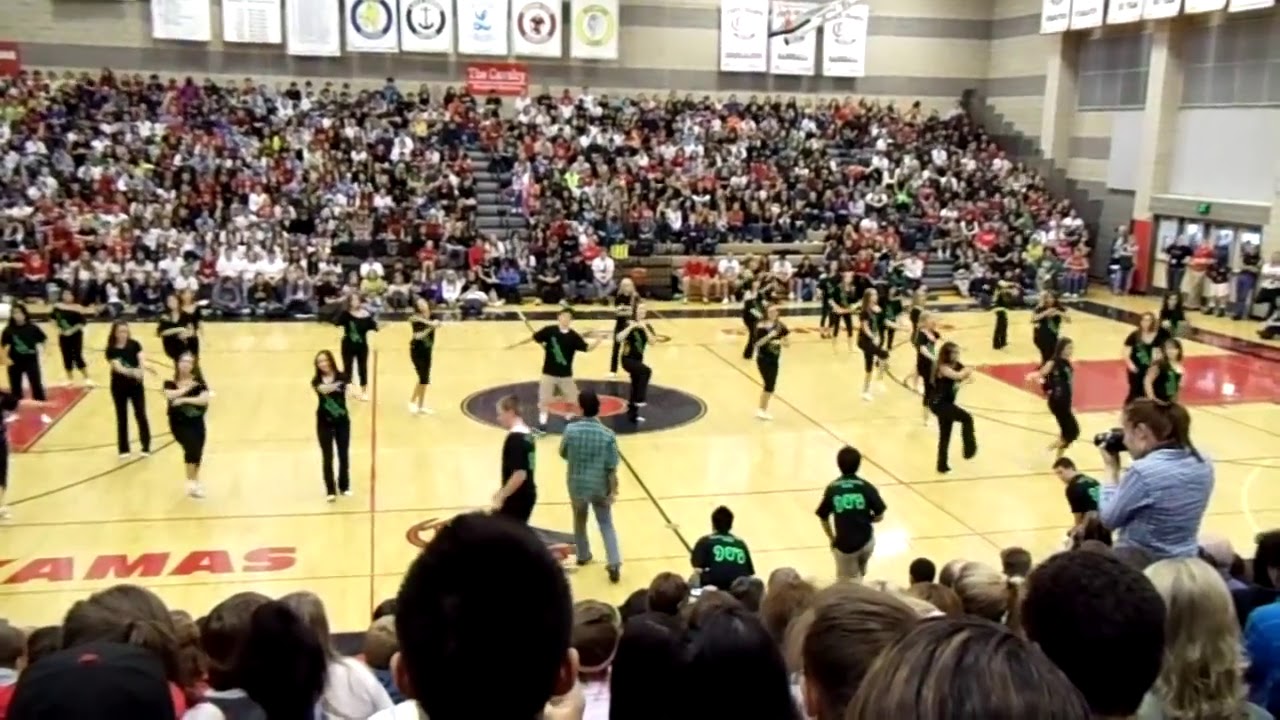The image captures a lively scene inside a high school gymnasium during what appears to be a pep rally or school event. The focal point is a group of approximately 20-25 students, both male and female, wearing predominantly black outfits, with a few boys in khaki shorts. They are engaged in a synchronized dance routine, with some raising one leg while others have their arms positioned variously at their sides or near their chests. The gym floor is yellow with black and red logos, and prominently features red letters spelling out something like "AMAS." Surrounding the dancers, the bleachers are densely packed with spectators, stretching up about 20-25 rows. The photo was taken by someone seated roughly 8-10 rows up, evident by the heads of people in the foreground. Additionally, a person in a blue shirt can be seen standing and using a digital camera to capture the event. The gym is adorned with banners celebrating various school championships and achievements, adding to the spirited atmosphere of the event.